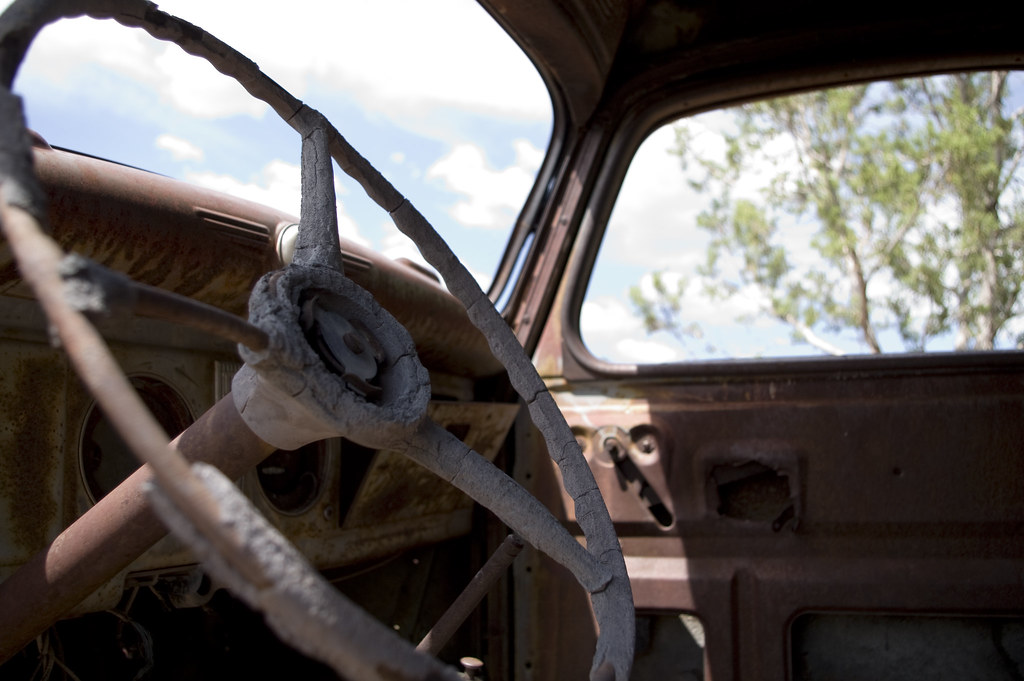This horizontally rectangular image captures the view from inside a dilapidated vehicle, looking outward from the driver's side. The vantage point is slightly angled upwards, as though we are seated in the driver's seat, gazing toward the confluence of the windshield and the passenger side window. The windshield reveals a bright blue sky adorned with heavy white clouds, while the passenger window frames a slender tree with sparse green leaves, set against the same vivid sky. The vehicle's interior is stripped down, exposing the raw, dark brown metal framework of the passenger door. On the left side of the image, the steering wheel is prominently displayed in a state of severe disrepair. Its original covering is brittle, cracked, and missing in patches, exposing the dark brown metal core beneath.